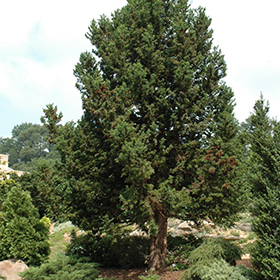This photograph captures a serene outdoor landscape dominated by a majestic deciduous tree, possibly an oak or maple, with a thick trunk standing prominently in the middle. Surrounding this central tree, there is a mix of other flora, including evergreen trees, which might be cedar or Lombardi poplars, and lower evergreen bushes framing the scene. The ground around the main tree is adorned with bushes, possibly forming a flowerbed, and scattered rocks, adding to the picturesque setting. The sky above is mostly white with hints of blue, indicating a partly cloudy day with sunlight softly illuminating the scene from the upper right, casting shadows to the left. This well-landscaped area, which could be someone's backyard or a rest area, is complemented by the presence of additional trees and the distant view of hills, creating a beautiful and tranquil atmosphere.